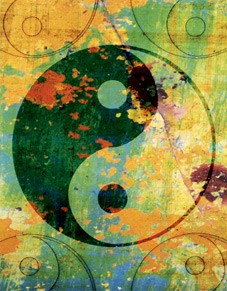This abstract graphic image intricately showcases the yin-yang symbol at its center, rendered in black and white with the classic opposing dots. The yin-yang, housed within a circular pattern, features splotches in both black and white sections, adding a contemporary twist to the traditional design. The surrounding background is vibrant and dynamic, pulsating with an explosion of colors—gold, green, blue, orange, yellow, purple, and reds—merging together in a splatter-painted aesthetic reminiscent of hippie art. Swirls of these hues intermingle, creating a fluid, almost melted appearance. Smaller circles adorn each corner of the image, and intricate circle designs are interspersed throughout, enhancing the overall complexity. The artistic arrangement of watercolors and blotches emphasizes the image’s creative and free-spirited nature.